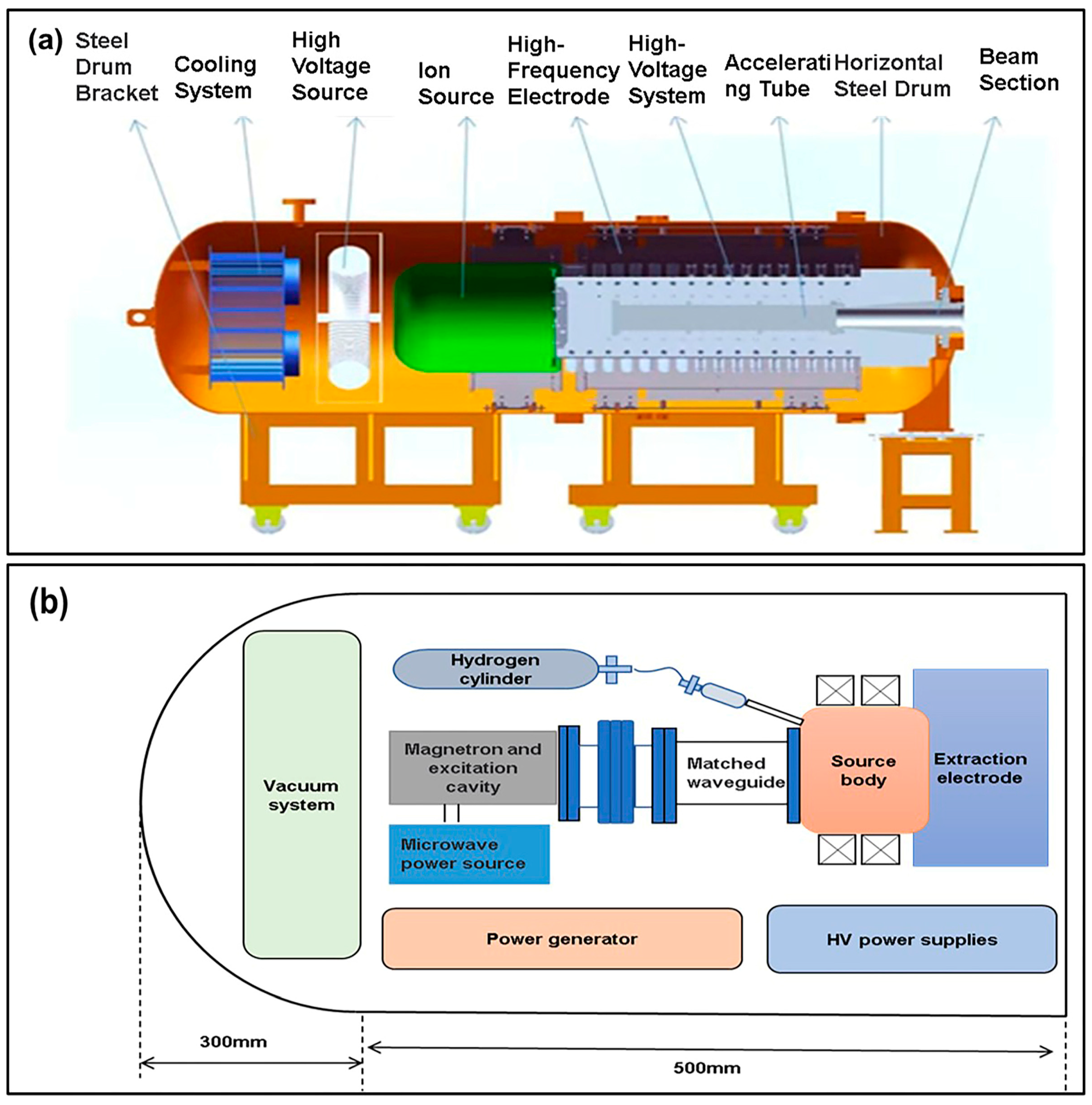The image is a detailed, two-part diagram labeled A and B, each representing different systems within cylindrical structures. 

In diagram A, a long, horizontal cylindrical tank, orange in color, lies on a steel drum bracket that serves as its frame. We see a cross-section of the tank with clear labels indicating its internal components, progressing from left to right. Starting on the left, there is a steel drum bracket, followed by a blue cooling system. Next, a white upright cylinder is labeled as the high-voltage source, adjacent to a green cylinder identified as the ion source. Further to the right, a series of gray, nested cylindrical components are marked with labels such as high-frequency electrode, high-voltage system, accelerating tube, horizontal steel drum, and beam section.

Diagram B, by contrast, features a more schematic representation, resembling a bullet shape with a rounded left end and a tapered right end. Internally, several components are depicted with colored rectangles and ovals. On the far left, a skinny green vertical rectangle is labeled as the vacuum system. Moving right, a gray oval labeled hydrogen cylinder connects via a cord and hose to a central source body. Below the hydrogen cylinder, within a blue rectangle, is the magnetron and excitation cavity. Adjacent to this is the microwave power source, encased in a bright blue box, followed by a peach-colored box labeled power generator, which sits below the HV power supplies. The source body also connects to components marked extraction electrode and matched waveguide. The entire bullet-shaped figure includes measurements indicating that it is 300 millimeters in length from the vacuum system to the tapered end and an additional 500 millimeters beyond that point to the end of the cylinder.

Both parts of the diagram use contrasting colors and are highly detailed, with diagram A providing a more realistic, colorful rendition, while diagram B is more schematic and utilizes color primarily for differentiation of components.